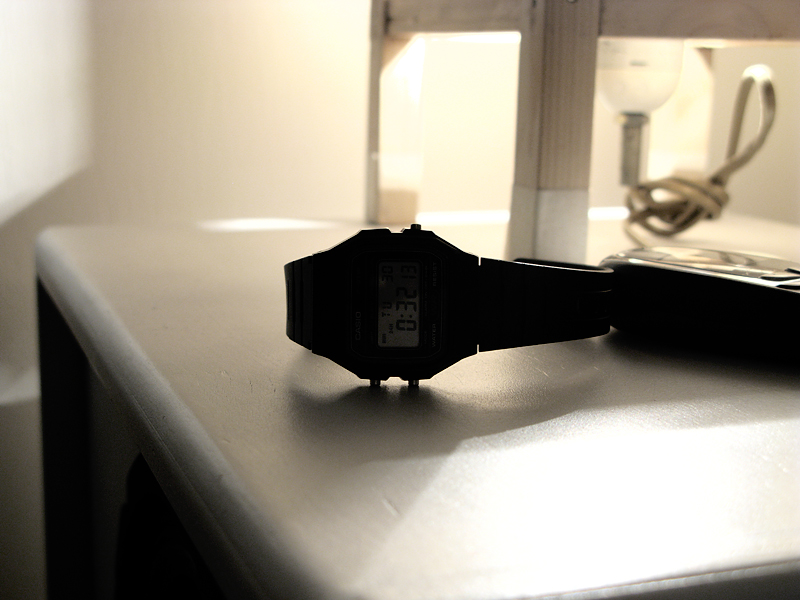In the image, a digital watch rests on a white-topped piece of furniture, possibly a nightstand or vanity. A light sconce is visible on the wall, its reflection caught in a nearby mirror. An electrical cord is neatly wound beside the watch. Next to the watch lies a black object, likely a flip phone, though the dim lighting makes it difficult to be certain. The walls are painted white, and the floor is not visible in the frame.